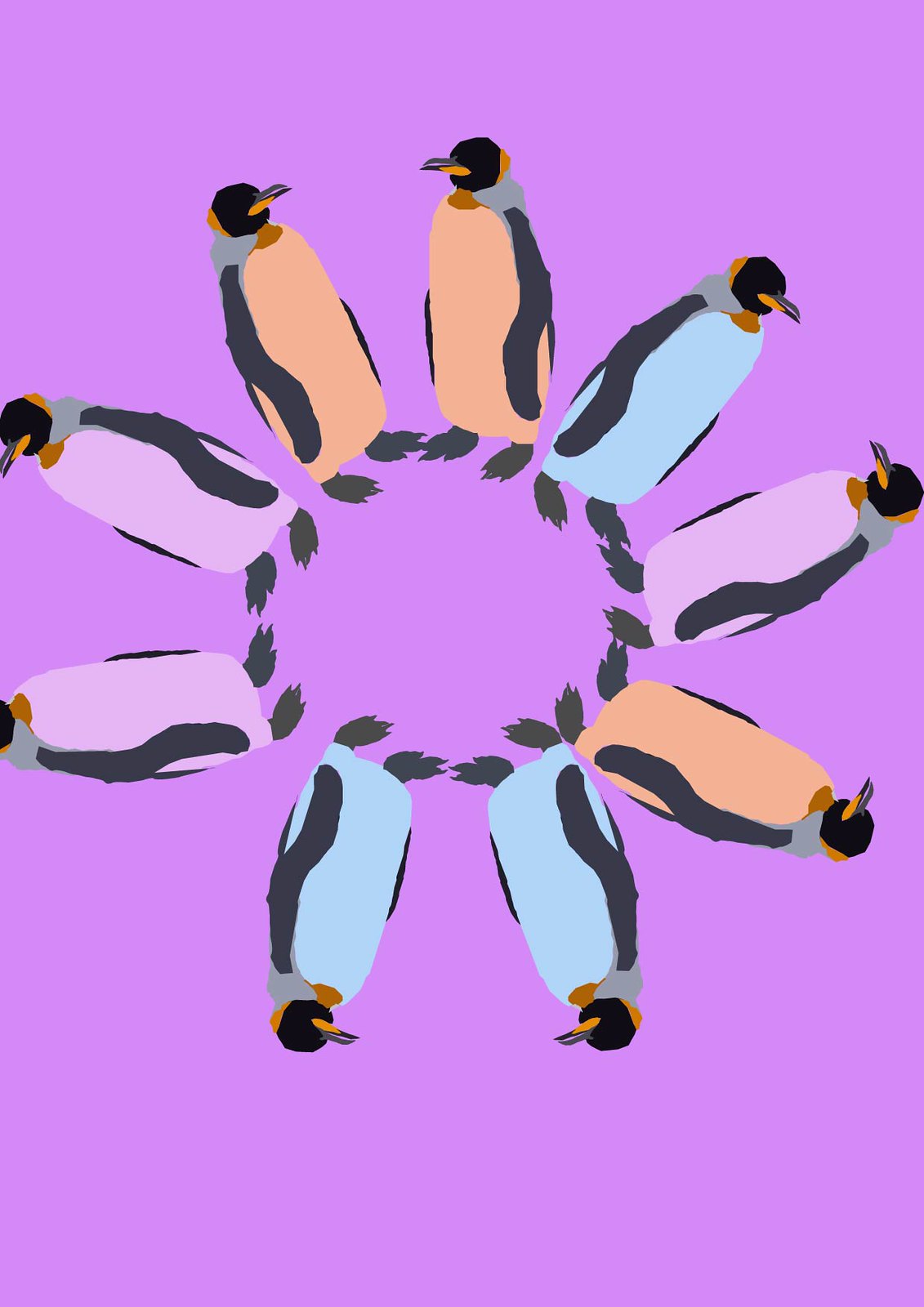The image depicts a vibrant pop art piece featuring a whimsical arrangement of nine penguins. The penguins are strategically positioned in a circle, resembling a flower with their feet pointing inward. This creates a visually engaging formation where the lower penguins appear upside down. The top two penguins showcase black wings, and heads with orange and black beaks, complemented by orange bellies. Moving clockwise, the next pair includes a light blue-bellied penguin on the right and a light pink-bellied penguin on the left, both consistent in their black and orange facial features. Another penguin to the right features a light gray body, while further along the circle, we encounter two penguins with pink bodies and light gray shoulders. Following them are two blue-bodied penguins with similar markings, one with a more muted pale green hue. The final penguin, part of a pair with an orange belly, faces outward, distinguishing itself from the others. Notably, one penguin's head is partially cropped due to the picture's framing. All penguins have striking black feet positioned against a soothing lilac background, which covers about three-quarters of the artwork. This creative and cute arrangement presents a dynamic visual feast in a delightful pop art style.